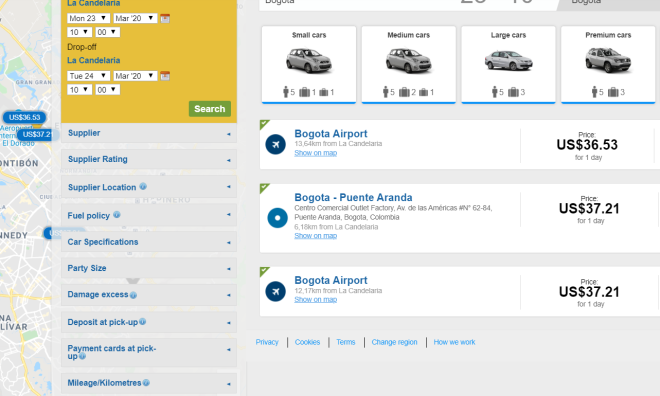This image is a screenshot of a car rental website. Prominently featured at the upper left is a distinctive yellow box where users can input their desired pick-up and drop-off dates, along with a search bar for convenience. Adjacent to the yellow box is a partial view of a map, providing geographical context. Below this input section, the interface lists various categories in blue text: these include 'Supplier,' 'Supplier Rating,' 'Supplier Location,' 'Vehicle Policy,' 'Car Specifications,' 'Party Size,' 'Damage Excess,' 'Deposit at Pick-up,' 'Payment Cards at Pick-up,' and 'Mileage/Kilometer.' Each category appears to be clickable for further details.

On the upper right, the website showcases four distinct boxes, each featuring an image of a car categorized as 'Small Cars,' 'Medium Cars,' 'Large Cars,' and 'Premium Cars.' 

Further down, the site displays specific rental listings in blue text within white rectangles. These listings include:
- "Bogota Airport" at a price of US $36.53
- "Bogota Puente Aranda" at a price of US $37.21
- Another listing for "Bogota Airport" at a price of US $37.21 

These elements come together to provide a detailed overview of car rental options available at different locations and price points.